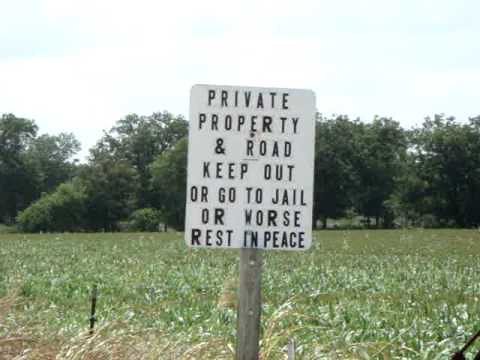In this outdoor landscape photograph, a gray wooden post supports a white rectangular sign with rounded corners displaying a warning in black print: "Private property and road. Keep out or go to jail, or worse, rest in peace." The foreground is occupied by a golden-colored patch of wheat, transitioning into a stretch of green grass that extends to a tall tree line with dark green foliage. The sky above is a very light, almost white blue, indicative of an overcast day. A small barbed wire fence marks the edge of the field, and there are a couple of short vertical dark stakes further in the background. The overall scene has an ominous tone, underscored by the sign's stark warning.